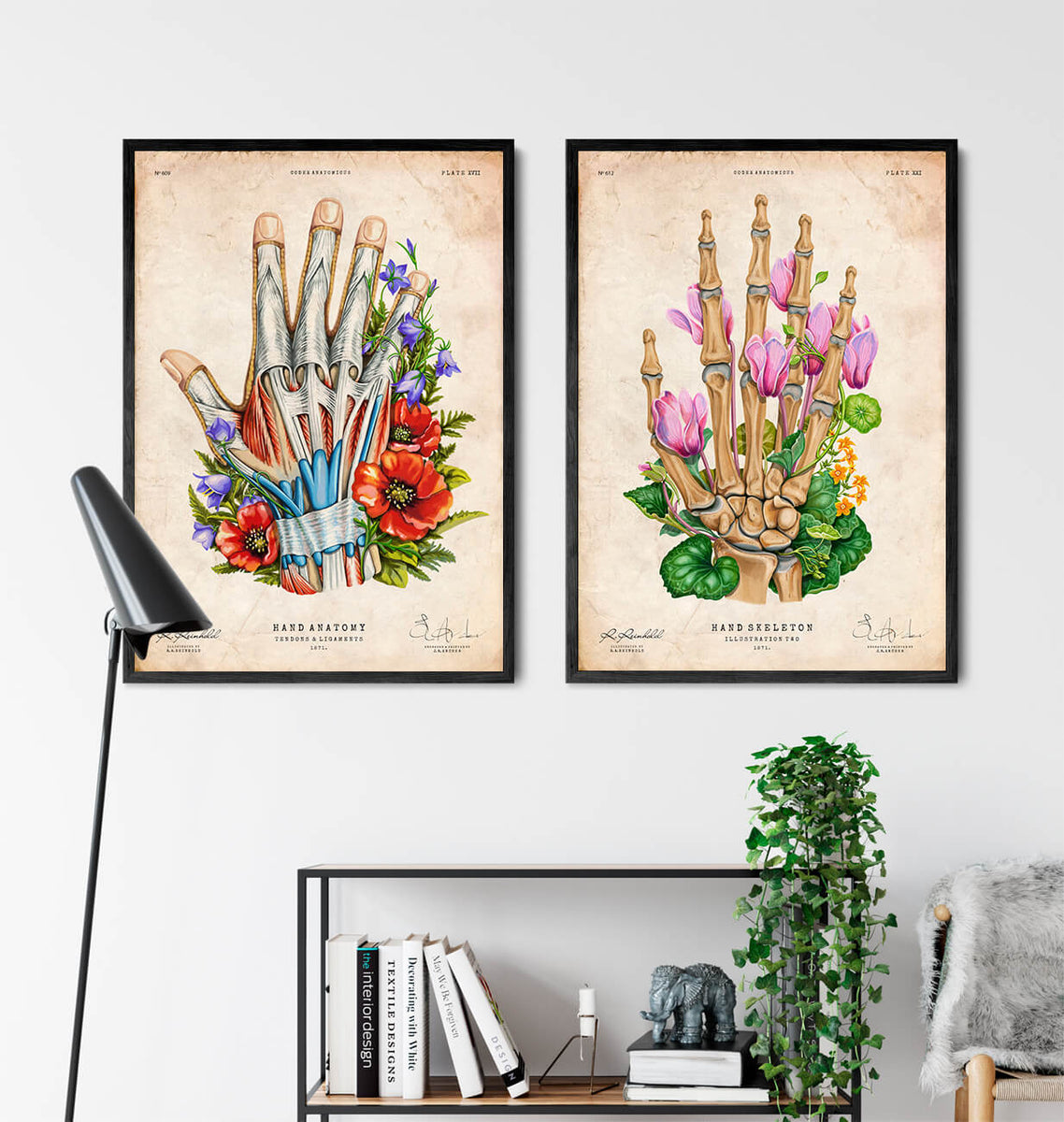The image depicts an indoor scene, likely a waiting room, characterized by a well-organized and aesthetically curated space. The focal point is a white wall adorned with two large, rectangular framed prints, each bordered by a small black frame and set against a light brown, parchment-like background. 

The print on the left showcases the anatomical intricacies of a hand, illustrating tendons and ligaments, with vibrant purple, red, and blue flowers intertwined around the fingers. Beneath this illustration, the label reads "Hand Anatomy."

The print on the right displays the skeletal structure of a hand, emphasizing the bones, and is adorned with green leaves and pink alongside gold flowers around the base. This print is labeled "Hand Skeleton."

Below these prints, a sleek black-framed shelf features an arrangement of white hardcover books, an elegant carved gray elephant figurine, and a gently cascading ivy plant in a pot. To the left of the shelf stands a tall, dark gray lamp with a matching lampshade. To the right, a wicker chair is draped with a light gray, faux fur throw, adding a touch of comfort and warmth to the room's decor.